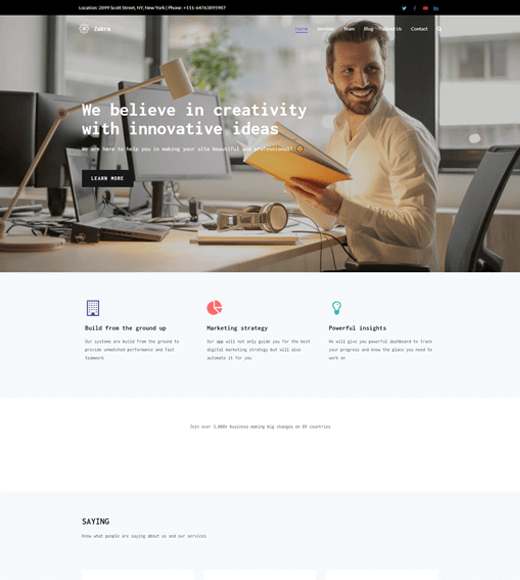Screenshot of Website Featuring a Tech Startup Theme

The image captures an entire webpage displaying a tech startup ambiance, albeit in a small, somewhat hard-to-read format. Dominating the top of the page is a large header image showcasing a Caucasian male with light brown hair and a beard, wearing a white button-up shirt. He is seated at a sleek, modern desk, surrounded by multiple monitors and laptops, accompanied by a tangle of wires that lend an authentic tech startup feel to the setting. Amidst the high-tech equipment, a pair of headphones rests casually atop a notebook, adding to the workspace clutter. The man is depicted smiling, looking to his right, while flipping through a book, exuding a blend of professionalism and approachability.

Above the header image, a black navigation bar houses social media icons, presumably for Twitter, Facebook, YouTube, and LinkedIn, in that order. The text within this bar is too small to decipher but likely includes contact details, possibly an address and phone number. The company name, "Zakra" (Z-A-K-R-A), is prominently visible.

Within the header image, purple and white menu options are displayed, though only the white text is legible, listing services such as "Services," "Teams," "Blog," "About Us," and "Contact." An inspirational slogan, "We believe in creativity with innovative ideas," is also featured within the header. A black call-to-action button with the text "Learn More" encourages user engagement.

Below the header, the layout transitions into three rows of infographics, each containing headers and accompanying text that are unfortunately too small to read clearly. These sections alternate in background color between white and gray, featuring black text, creating a visually appealing and structured design that suggests an organized presentation of information.

Overall, the webpage exudes a modern, innovative vibe typical of a contemporary tech startup, with an emphasis on creativity, innovative ideas, and accessibility to various services and information through a well-organized interface.